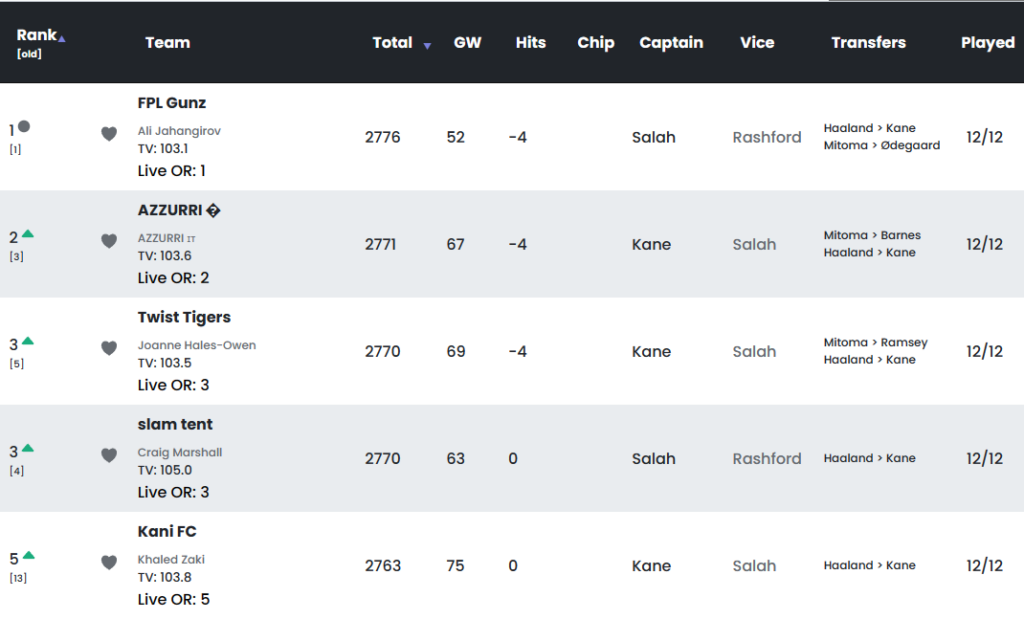In the image, the background features alternating blue and white stripes. At the top of the image, there's a black box containing columns that label various stats: "Rank," "Old" (denoted in parentheses), "Team," "Total" (accompanied by a blue down arrow), "GW," "K," "D," "Chip," "Captain," "Vice," "Transfers," and "Played."

Below these headings, the first row is set against a white background and labeled "FPL Guns" with a heart icon. It shows the following data: 
- Rank: 2776
- Total: 52
- Transfers: -4
- Captain: Salah
- Vice-Captain: Rashford
- Played: 12 out of 12

The next row sits on a blue background labeled "Azura," also marked with a heart and a diamond shape. It lists:
- Rank: 2771
- Total: 67
- Transfers: -4
- Captain: Kane
- Vice-Captain: Salah
- Played: 12 out of 12

Third, on a white background, labeled "Twist Tigers" with a heart icon:
- Rank: 2770
- Total: 69
- Transfers: -4
- Captain: Kane
- Vice-Captain: Salah
- Played: 12 out of 12

The next row, on blue, labeled "Slam Tent" with a heart icon, provides:
- Rank: 2770
- Total: 63
- Transfers: 0 hits
- Captain: Salah
- Vice-Captain: Rashford
- Played: 12 out of 12

Finally, the last row on a white background is labeled "Kenny FC" accompanied by a heart icon:
- Rank: 2763
- Total: 75 
- Transfers: 0 hits
- Captain: Kane 
- Vice-Captain: Salah 
- Played: 12 out of 12